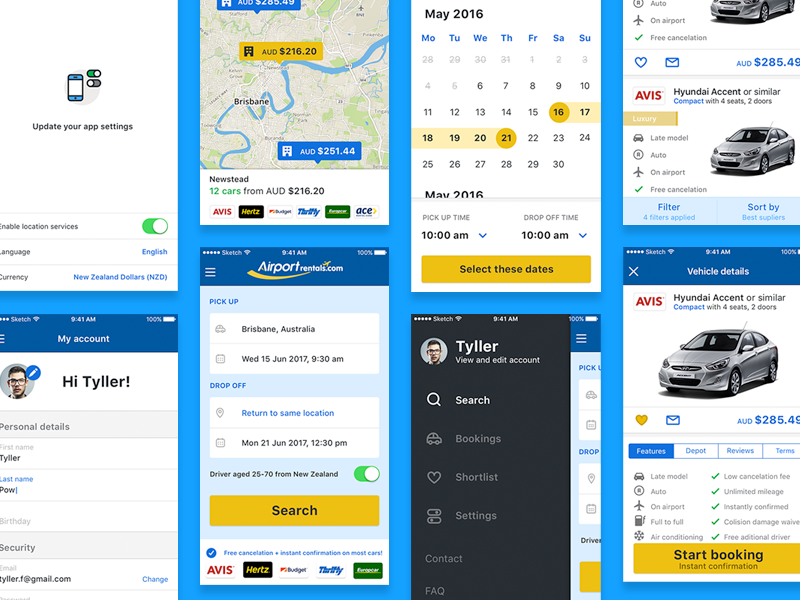Tyler's iPhone screen displays several distinct pages, each meticulously captured and shown individually. The primary page prompts the user to update their app settings, with the 'Enable Location Services' option visibly activated. The system language is set to English, and the currency preference is New Zealand dollars.

Another screen focuses on rental vehicles, showcasing options from well-known companies like Avis and Hertz. Specifically, there are mentions of multiple Hyundai Accent models or similar vehicles, indicating that Tyler has been reviewing and considering these rental choices.

Additionally, one page is dedicated to an airport rental service, airportrentals.com. It details a reservation for a trip starting in Brisbane, Australia. The pick-up is scheduled for Wednesday, June 15, 2017, at 9:30 a.m., and the drop-off is set for Monday, June 21, 2017, at 12:30 p.m. This collection of separate yet related pages provides a comprehensive view of Tyler's detailed planning process for an upcoming trip.